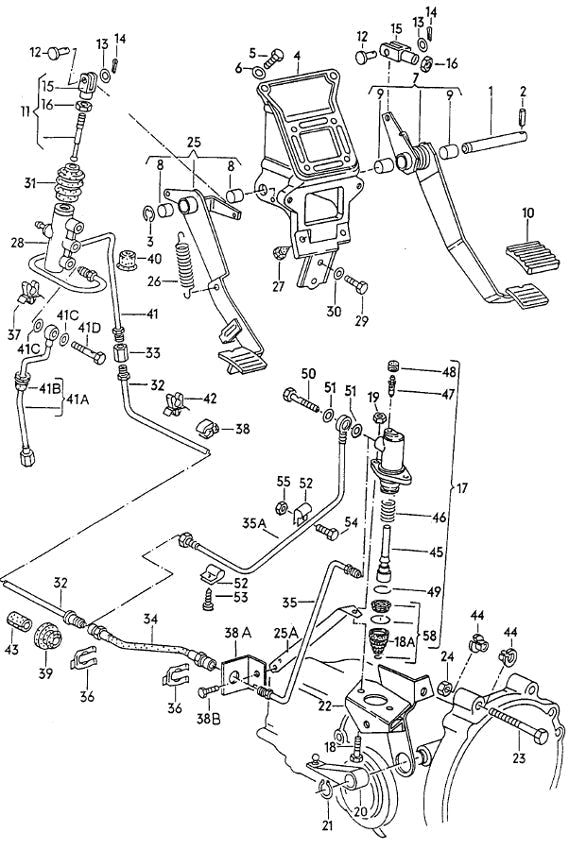The image is a detailed black-and-white schematic from an instruction manual for assembling a complex piece of machinery. The manual features a plethora of parts including bolts, nuts, screws, and possibly foot pedals, all meticulously numbered with a combination of numbers and letters, such as 12, 13, 41A, 41B, and up to 58. The background is entirely white, emphasizing the technical and mass-produced nature of the diagram. The parts vary in size and shape, some are minute like screws and pins, while others appear larger and more complicated. This comprehensive diagram lacks a border and a key, making it challenging to discern the specific nature or final form of the assembled item solely from this image.